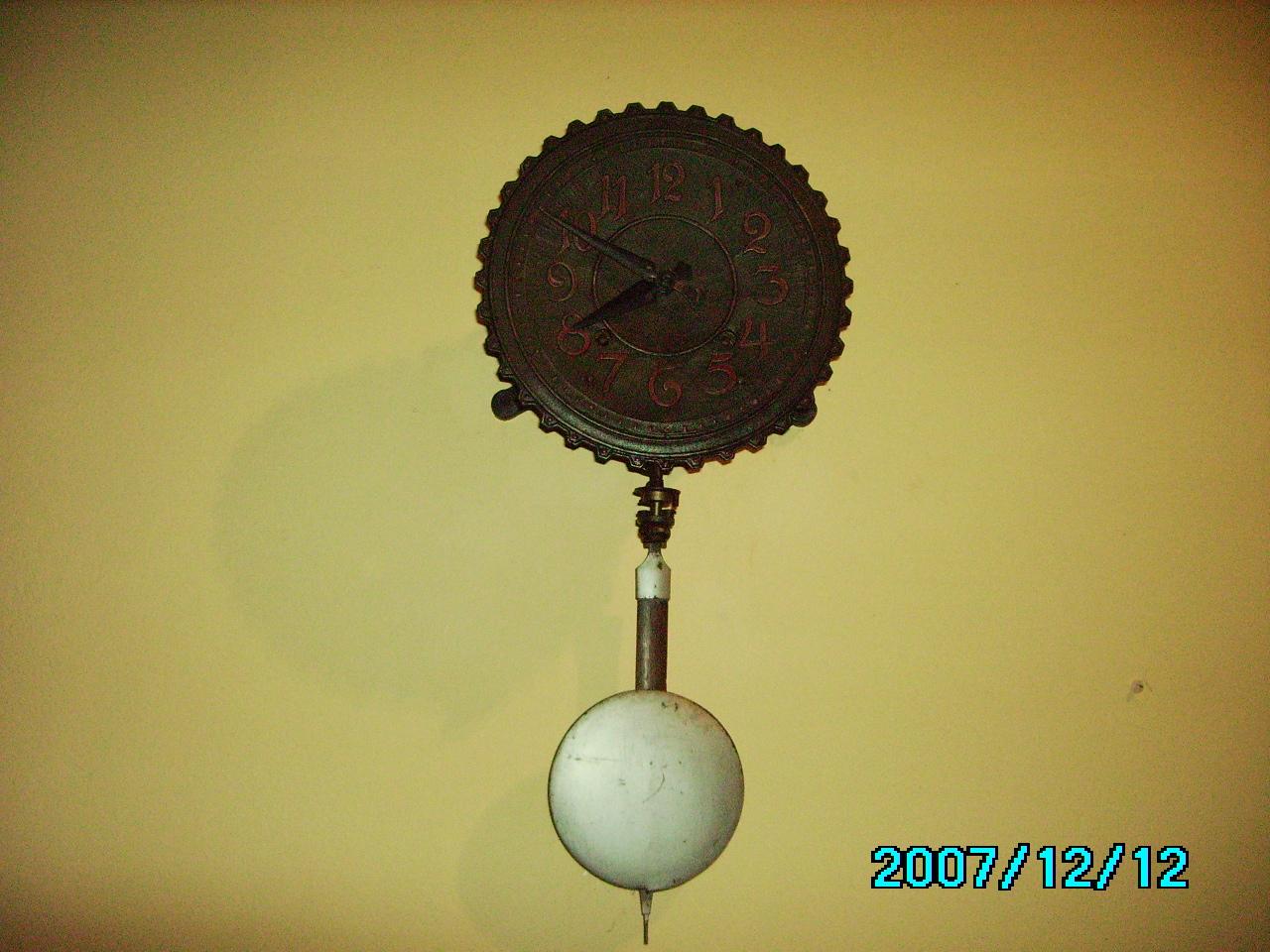Caption: 

The photograph captures a vintage wall-mounted clock characterized by its metallic face, which bears a weathered, bronze-like appearance. The clock features a flat surface accented by ridges along its perimeter, resembling the form of a dial. The inner section of the clock showcases hour markings in a dark red hue, while the clock's hands are a stark black, providing a subtle yet striking contrast. Suspended from the clock is a slender metal arm that culminates in a prominent, silver medallion, likely a pendulum that oscillates to mark the passage of time. The clock indicates the time as 7:50, and a small date display on the bottom right reads December 12, 2007. An informative website, www.FEMA.gov, is referenced at the bottom of the photograph.